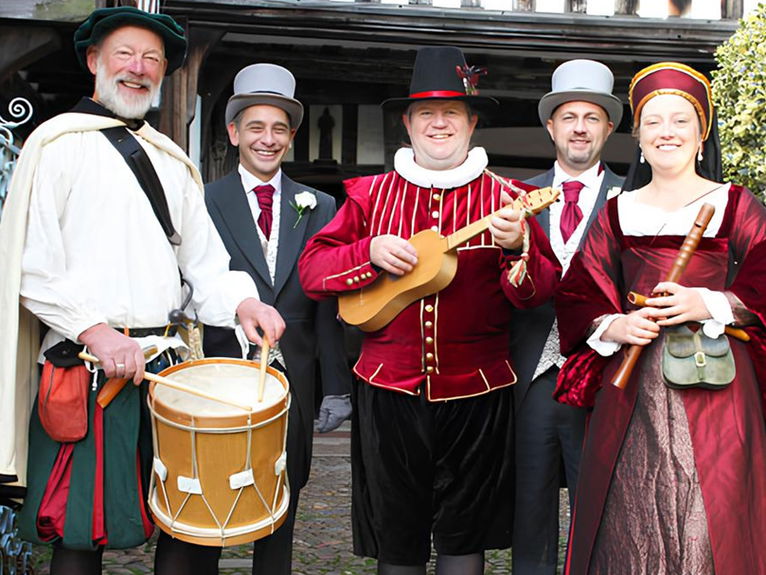In this color photograph, a lively scene unfolds at a wedding, featuring a historical reenactment with five individuals—four men and one woman—dressed in old-fashioned attire. The backdrop includes a building with brown wooden trim and a tree in the upper right-hand corner. On the left side, a cheerful drummer wearing a white shirt, a green and red pleated skirt, and a green hat stands out with his old-time drum secured by ropes. Next to him, a man in a darker gray suit, top hat, gray gloves, and red tie adds to the vintage aesthetic. Following him, another man wears a fanciful outfit consisting of a black hat, a red long-sleeve shirt with a distinctive, playing card-like collar, velvet black shorts, and black tights. The central figure, dressed in a gray suit similar to the man with the top hat, is playing a small lute or ukulele. Completing the ensemble is a woman in a radiant, silky red dress and matching head covering, playing a brown wooden flute. The composition suggests a historical or fantasy-themed wedding, enriched by vivid hues of dark green, beige, red, and black, though the lighting and shadows cast an edited, surreal quality over the image.